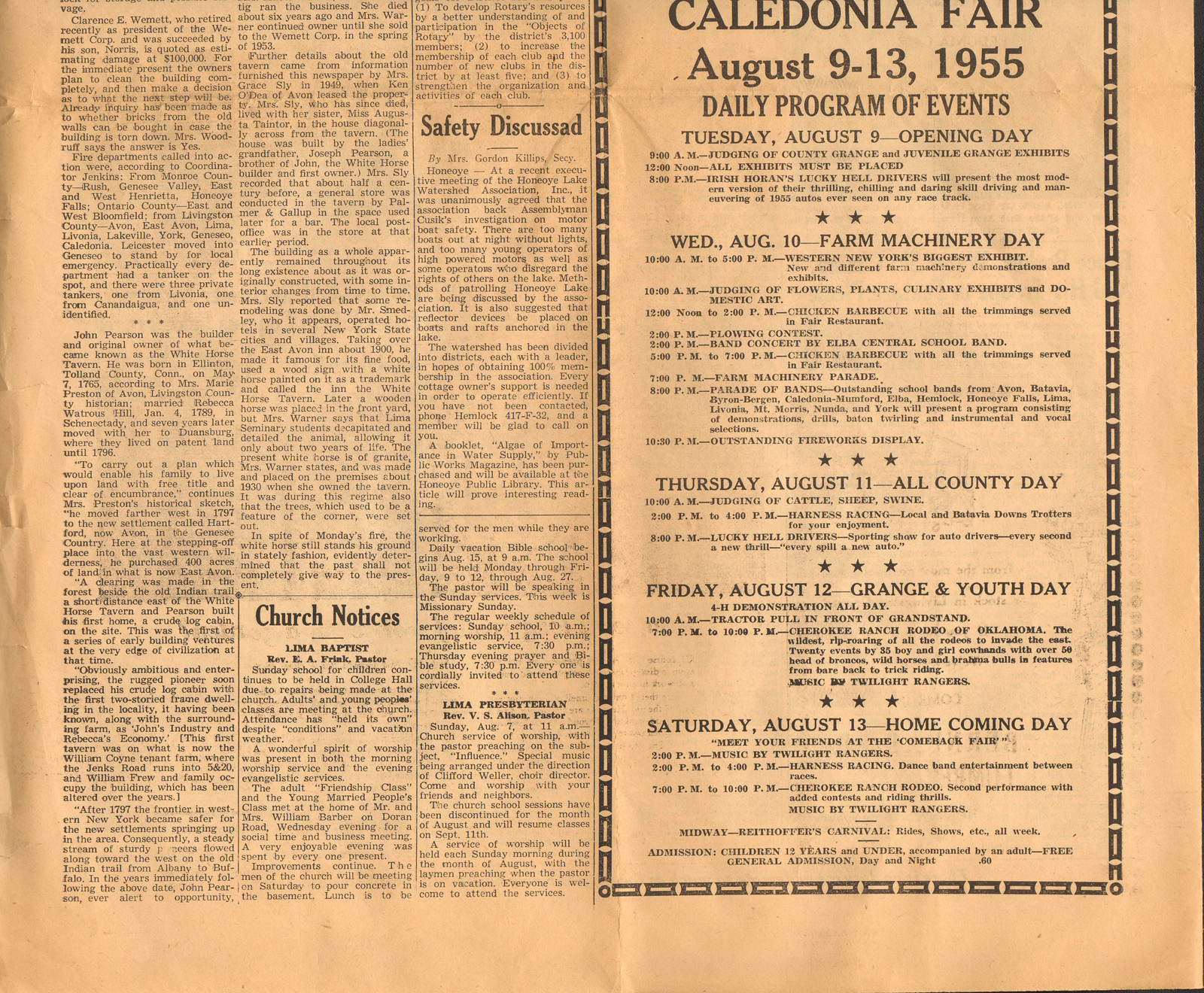This black-and-white newspaper clipping, slightly wrinkled and creased with a faint sepia tone, is divided into two sections. The left side features three columns of text with bold subheadings such as "Safety Discussed" near the top of the right column, "Church Notices" halfway down the center column, and mentions of "Lima Presbyterian" and "Lima Baptist" toward the bottom. The text in these columns is small and difficult to read due to the age of the paper.

On the right side, framed by a border of long black rectangles in a chain pattern, is a detailed display ad for the Caledonia Fair, held from August 9th to 13th, 1955. The ad outlines the daily program of events: Tuesday, August 9th, is the Opening Day; Wednesday, August 10th, is Farm Machinery Day; Thursday, August 11th, is All County Day; Friday, August 12th, is Grange and Youth Day; and Saturday, August 13th, is Homecoming Day. Each day’s listing is separated by three stars, and the font is small but legible, maintaining the vintage style of mid-20th century newspaper design.